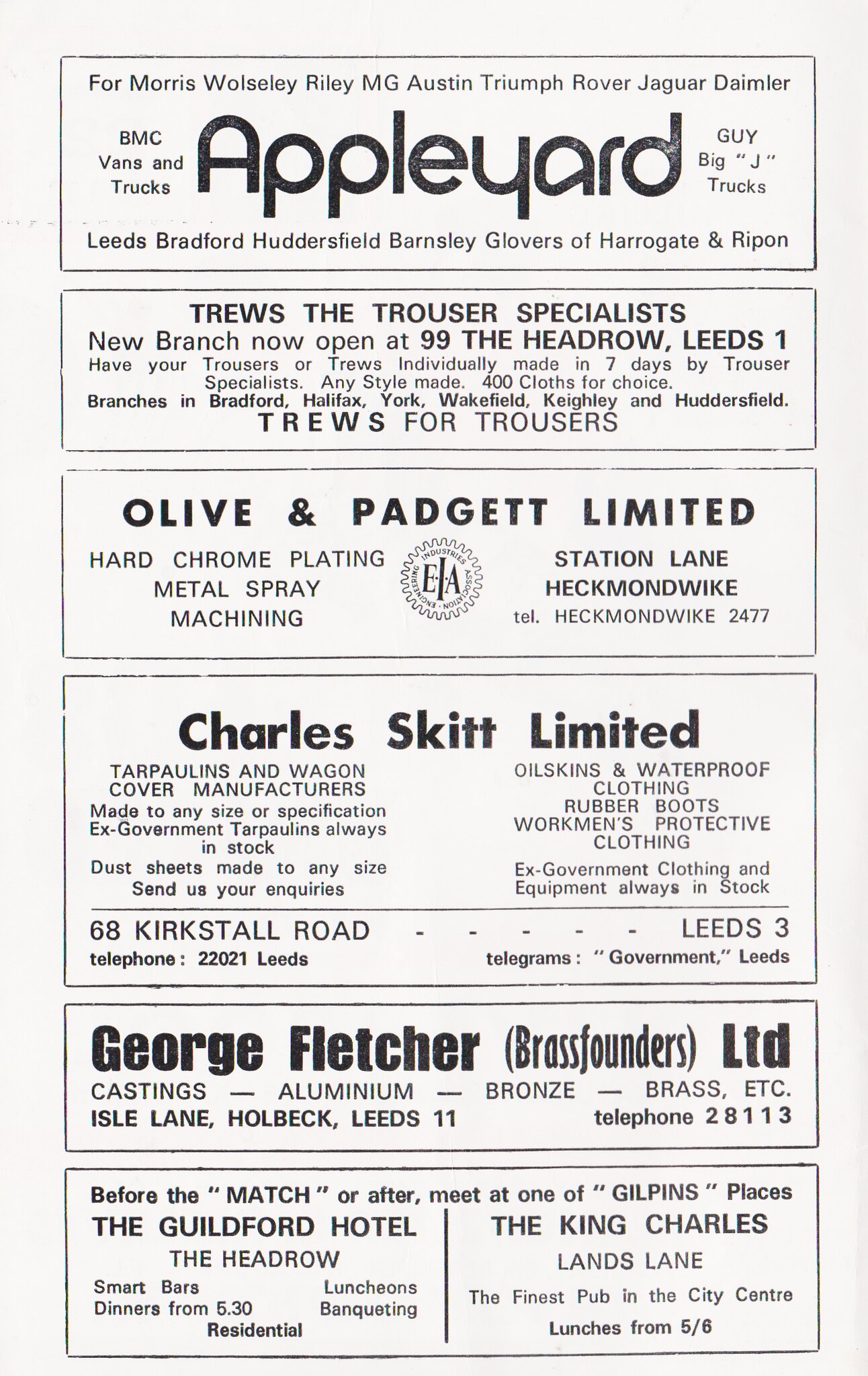This black-and-white image resembles a magazine page filled with various rectangular advertisements for different services and locations. At the top, there's an ad for Apple Yard, listing automotive brands like Morris, Wellesley, Riley, M.G., Austin, Triumph, Rover, and Jaguar, along with BMC vans and trucks. The service areas mentioned include Leeds, Bradford, and Huddersfield, with Glover's locations in Harrogate and Ripon. 

The next section features "Trues, the Trouser Specialists," highlighting a new branch at 99 The Headrow, Leeds. It emphasizes custom-made trousers ready in seven days, with a selection of 400 fabrics. Other branches are listed in Bradford, Halifax, York, Wakefield, Keighley, and Huddersfield.

Following that is an advertisement for Olive and Padgett Limited, offering hard chrome plating and metal spray machining, based in Station Lane, Heckmondwike. The contact telephone number is Heckmondwike 2477.

Next, there is an ad for Charles Skitt Limited, detailing their tarpaulin and wagon cover manufacturing services, alongside their provision of ex-government tarpaulins, dust sheets, oilskins, waterproof clothing, rubber boots, and workman’s protective wear. The address given is 68 Kirkstall Road, Leeds, with a telegram contact labeled "Government, Leeds."

Below that, George Fletcher Brass Founders Limited advertises their services in casting aluminum, bronze, and brass, located at Holbeck, Leeds 11, with the phone number 28133.

At the bottom of the page, the ad suggests visiting one of the Gilpin's venues before or after a match, such as the Guildford Hotel, Pedro Smart Bars, or the King Charles on Land's Lane, promoting dining options including luncheons and banquets.